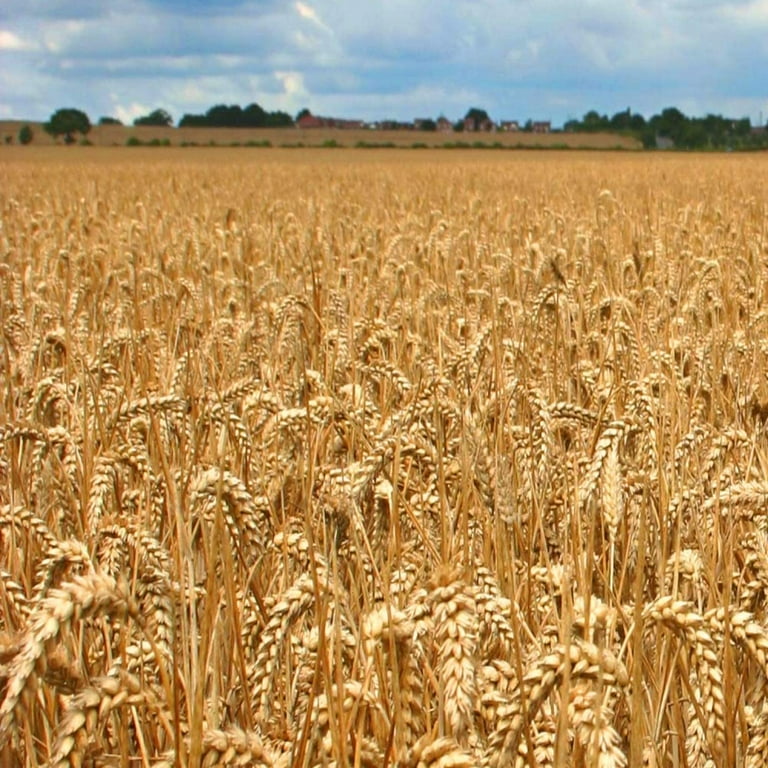The photograph captures an expansive wheat field stretching from the foreground, where individual golden blades of wheat are clear and in sharp focus, into the distance where they blur into a mass of indistinct vegetation. The field likely spans over an acre, leading up to a tree-lined horizon about seven-eighths of the way up the square-shaped image. Here, several additional farm structures can be discerned upon close inspection, suggesting an active farmland landscape. In the background, the sky is predominantly blue but beset with overcast clouds, with sunlight subtly illuminating portions of the sky, particularly on the upper left and right-hand corners. Just below the horizon in the upper right portion of the photograph, a farmhouse is faintly visible, nestled among the trees. The image’s simplicity and well-composed nature emphasize the vastness and serenity of the rural scene.